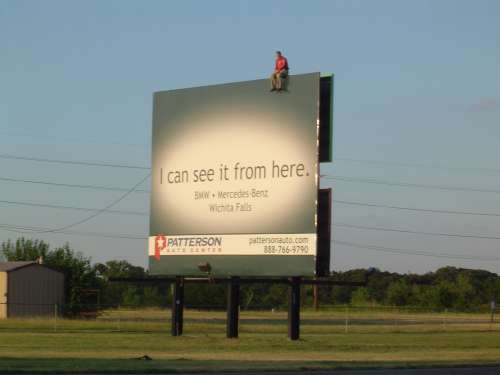This roadside billboard, located near Wichita Falls, is prominently featured against a backdrop of blue sky and a sparse landscape with green grass and trees. It's elevated on three evenly spaced black poles, and a chain-link fence runs parallel to the road just beneath it. The lower portion of the image reveals a small slice of the asphalt road.

The billboard itself is large and square, with a gray base and a central white section displaying bold black text that reads, "I can see it from here. BMW, Mercedes-Benz, Wichita Falls." Beneath this, a white banner with the partially legible text "Patterson Auto Center" appears blurry but discernible upon close inspection. To the right, an additional line includes the phone number 888-766-4790 and a website, PattersonAuto.com.

A distinctive feature of the billboard is the mannequin perched at the top right corner, dressed in a red shirt, khaki pants, and black shoes, mimicking a man casually sitting and gazing down at the viewer, adding a playful touch to the advertisement.

In the surrounding environment, a gray building with a blue top is visible to the left, partially obscured by the chain-link fence. Beyond this, a large green tree stretches across the background. Additionally, four power cables traverse the sky above and behind the billboard, enhancing the overall sense of depth and realism in the scene.